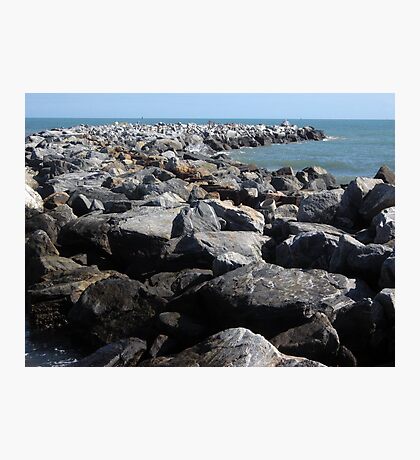This is a digitally enhanced photograph showcasing a coastal scene. The image has been neatly placed inside a display-holder with a grey background, indicating it has been cropped and refined. The primary focus of the photograph is a rugged, rocky shore composed of large, gray and black boulders. These rocks form a pier-like structure that extends towards the sea and displays a complex, almost spiral curvature. The rocks cover a significant portion of the image, dominating the foreground and central area. The ocean appears above the rocks, featuring a deep blue hue. Above the ocean, the sky occupies a thin strip at the top of the photograph, showcasing a light blue, cloudless expanse. The scene is bathed in daylight, as evidenced by the light reflecting off the rocks. No text is present on the image, ensuring the natural beauty of the setting remains uninterrupted.